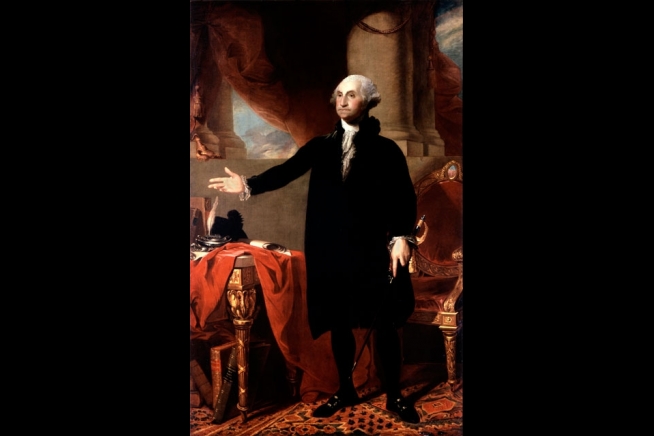The image is a vertically rectangular painting with large black borders on the left and right sides, occupying about one-third of the image each. In the central portion, there is an ornate portrait of George Washington. Washington is depicted standing elegantly in a black gown, contrasted by a white shirt and a white powdered wig. His left arm is extended outward, with a visible sword hanging in his right hand. Behind him is a luxurious, velvety red chair, resembling a throne. To his left, a wooden table is draped with a rich red cloth and adorned with scattered papers, a quill pen, and what seems to be books. In the upper left corner, there appears to be a window with a shade, framing the scene and revealing some cement columns in the background.